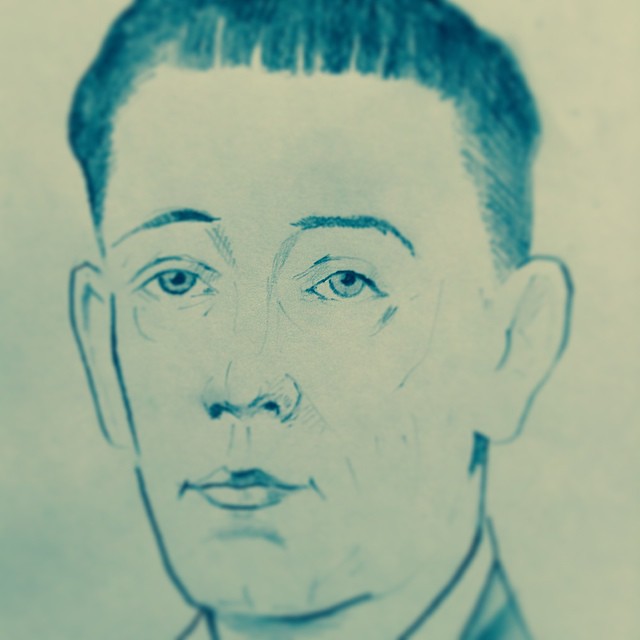The image is a hand-drawn illustration of a young Caucasian man’s face, likely scanned into a computer, rendered on a piece of beige, mustard-toned paper. The sketch, which some might see as done with charcoal or color pencils, emphasizes certain facial features more than others: the nose, lips, and eyes are highly detailed and in focus, while the right ear and hairline are slightly blurred, possibly due to the medium or the scanning process. His irises are intricately sketched, and his eyebrows, detailed nostrils, and subtle shading beneath his chin add to the realism. The man has a short haircut with a straight fringe across his forehead and appears to be wearing a suit, although only the collar and part of the shirt are visible as they drift out of the frame. His expression is thoughtful, perhaps even stoic, gazing directly at the viewer with restful, blue eyes and a hint of a wry smile. The artistic style and composition suggest it might be from the 1950s or 60s, capturing a moment of quiet introspection.